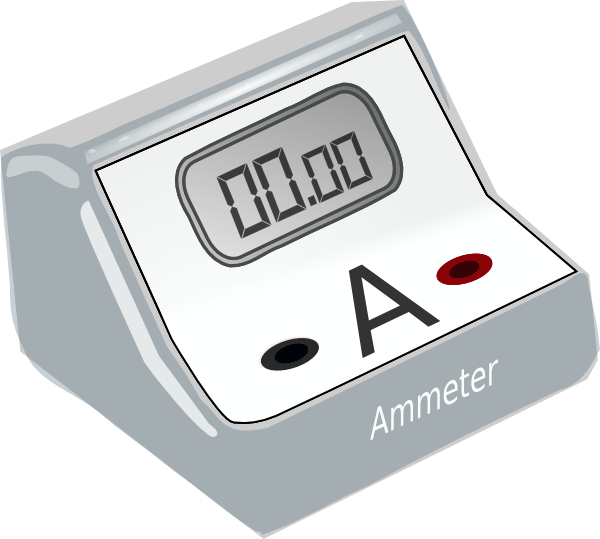This is a digitally produced image of an ammeter, rendered in a clip art style. The ammeter, which measures electrical current in amperes, is depicted as a gray square box with a front panel that dips inward. The front panel features a white area outlined in black, within which are a large black letter "A," a digital display reading "00.00," a black button to the left of the "A," and a red button to the right. Above the "A" is the digital display. This image is not a photograph but rather a computer-generated representation, likely created using software like Photoshop, serving as a demonstration of what an ammeter looks like. The background of the image is white. Ammeters, such as the one illustrated, are used to measure the flow of electricity in a circuit, helping homeowners determine if an outlet or an appliance is malfunctioning by checking if the electricity flow is as expected. This specific ammeter does not show an active reading, indicating it's not attached to any circuit in the representation.